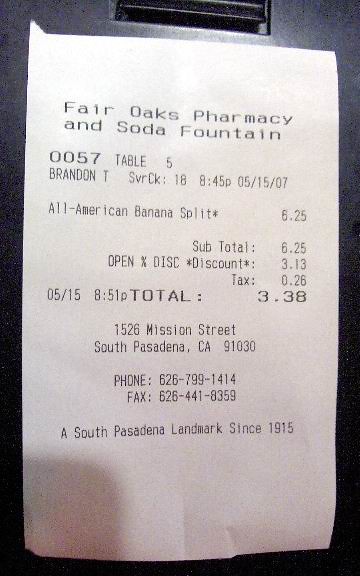In this snapshot, a receipt from Fair Oaks Pharmacy and Soda Fountain is prominently displayed against a black background. The receipt, printed on white paper, details a transaction handled by server 0057, Brandon T., at table 5. The date and time of the transaction are marked as 8:45 PM on May 15, 2007. The patron ordered an All-American Banana Split for $6.25. An open percent discount of $3.13 was applied, resulting in a subtotal of $3.12 with an additional $0.26 tax, bringing the grand total to $3.38. The address of the establishment is listed as 1526 Mission Street, South Pasadena, California, 91030, accompanied by the phone and fax numbers. At the bottom of the receipt, the motto "A South Pasadena Landmark Since 1915" is prominently featured. Notably, no tip appears to have been left for Brandon T.